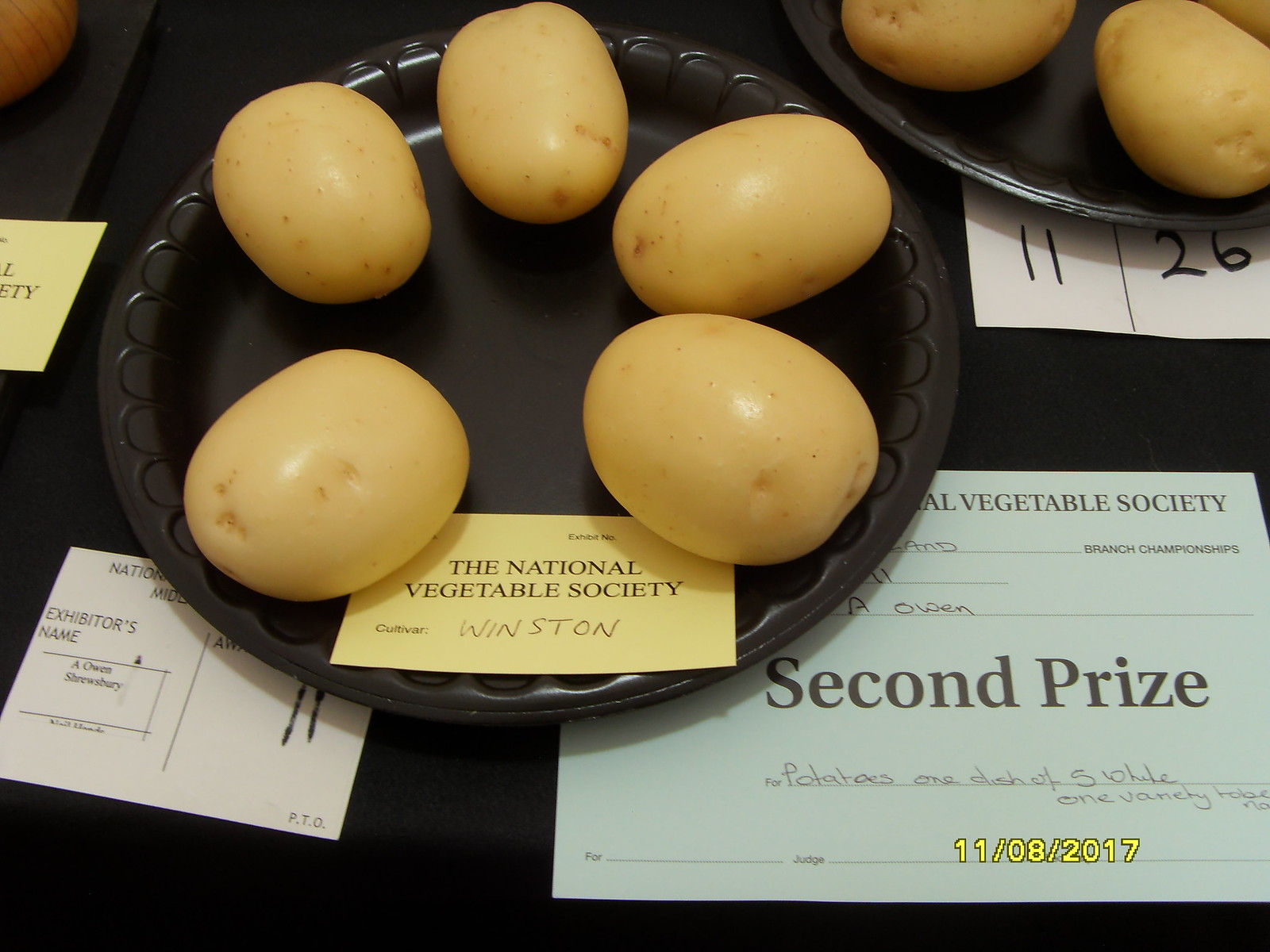The image depicts a black plate, likely made of plastic or foam, arranged on a table. Featured prominently on the plate are five clean potatoes with a thin, tan skin, meticulously organized around the edge. Beneath two of these potatoes is a light yellow card inscribed with "The National Vegetable Society," along with other details including "Cultivar" and the name "Winston" in pencil. Adjacent to the plate, partially visible, is a blue certificate creased under the plate, prominently labeled "Second Prize for potatoes, one dish of five, one variety," dated August 11, 2017. Surrounding the main focus, additional plates and vegetables, including what appear to be onions, are visible but partially cut off, indicating the broader context of a competitive event with various labeled entries.